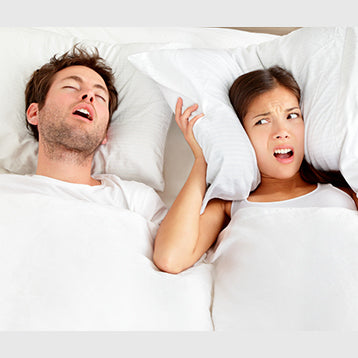The image depicts a white couple with brown hair lying flat in a bed under white bedding, which includes pillows, sheets, and a duvet. The background is similarly white, creating a monochromatic setting. On the left side, the man, who has a five o'clock shadow and is wearing a white t-shirt, is sleeping with his eyes closed and mouth open. On the right, the woman, dressed in a white tank top, has her eyes wide open, her mouth slightly ajar, and a clear expression of disgust or annoyance on her face. She is holding her pillow tightly against her ears, seemingly to block out the noise, suggesting that the man is snoring loudly. Both are positioned waist-up in the frame, emphasizing their contrasting reactions in this intimate setting.